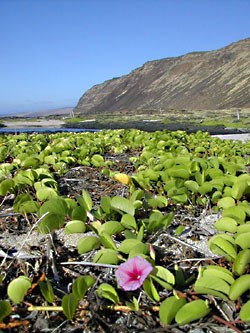This is a detailed portrait-oriented photograph taken outdoors, showcasing a natural setting. At the bottom of the image, a ground is covered with small green leaves of a plant, prominent in their lush greenery. In the very center at the bottom, a single, striking pink flower stands out, fully in bloom. The inner part of the flower is a deeper pink with a star-shaped pattern, while its outer petals are a lighter pink. The background of the photograph features a vast landscape with what seems to be a body of water or possibly an ocean stretching into the horizon. A grassy shoreline is visible, leading up to a large, rugged mountain that is brown to dark gray in color, devoid of vegetation. Above the mountain, the sky is clear and blue, adding a serene atmosphere to the scene. The image captures the essence of a bright, cloudless daytime environment.